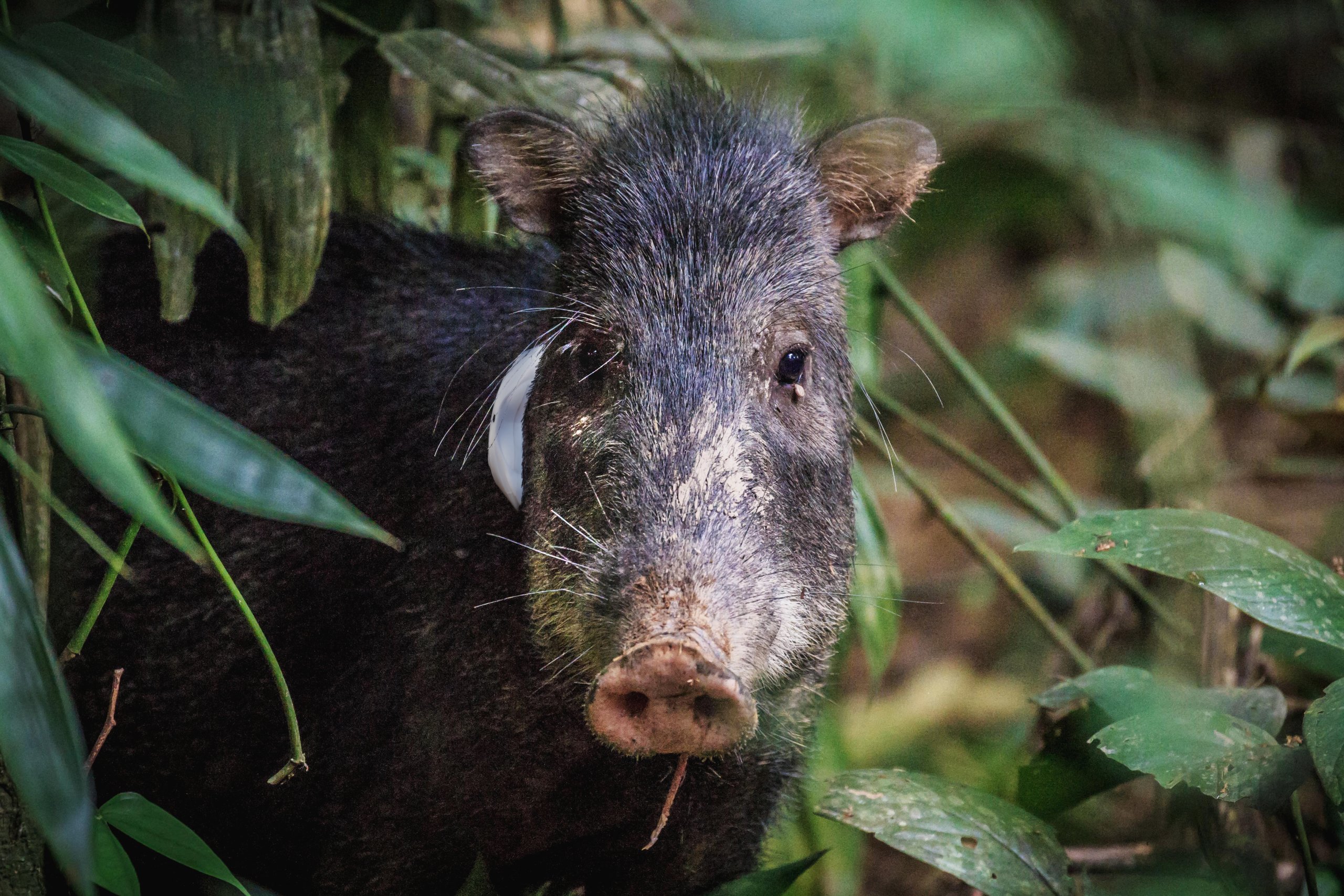In this rectangular, close-up photograph taken in the woods, the focal point is a young wild boar emerging from the left side of the image. The boar's face, turned forward, features an endearing pink snout surrounded by a narrow head. Dark eyes, partially obscured by a few stray whiskers and delicate eyebrow-like hairs, add to its expressive demeanor. Two small, almond-shaped ears top its head, which is also adorned with a tuft of coarse bristles. Notably, this young or possibly female wild boar lacks tusks, enhancing its gentle appearance. The lower left of the image captures a glimpse of its darker, brownish-black body. Surrounding the boar's head are lush, deep green leaves and branches, providing a natural frame that highlights the creature's sweet, inquisitive face.